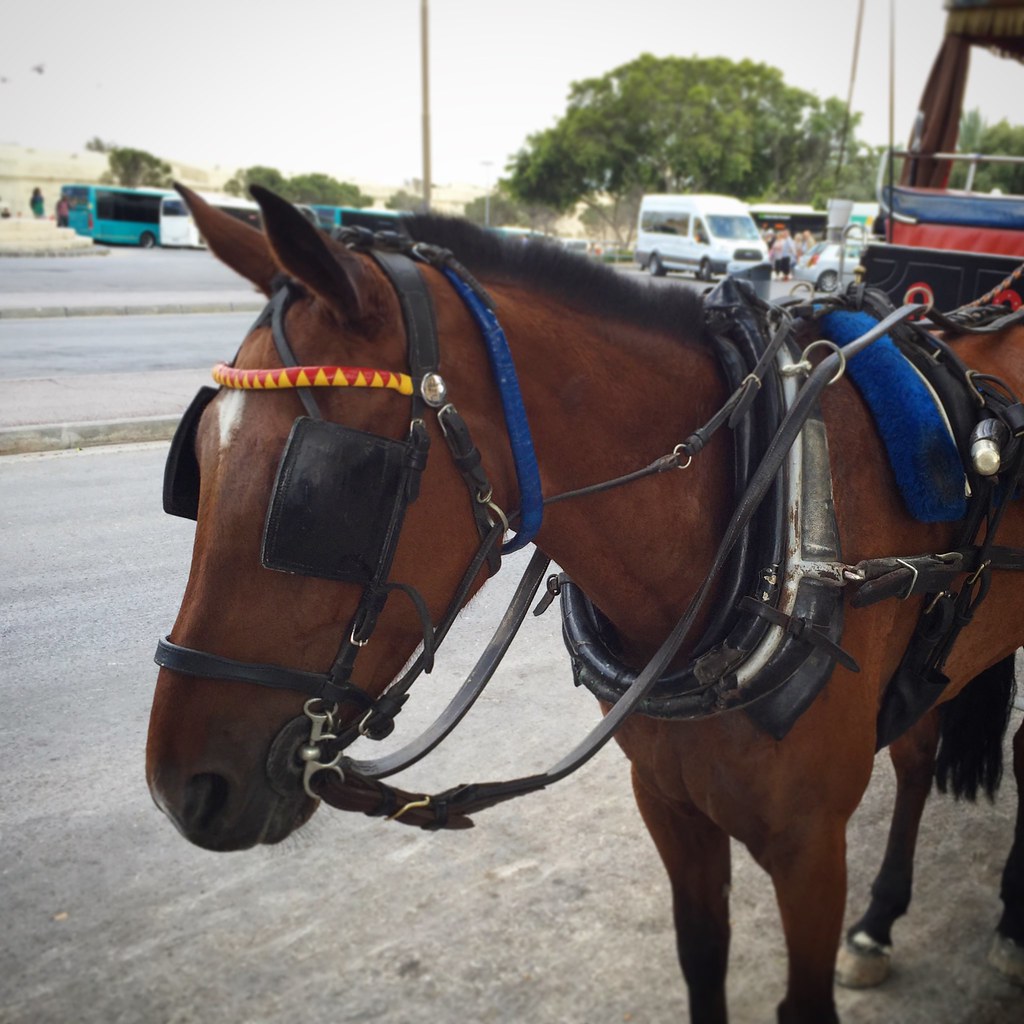In this detailed outdoor scene, a close-up of a bay horse with a black mane and a distinctive star on its forehead is the focus. The horse is harnessed and bridled, hinting at its attachment to a carriage or wagon, though the exact vehicle is obscured from view. Notably, it wears blinders—black square fabric pieces covering both eyes—adding an interesting element to its gear. The horse stands on a somewhat worn concrete surface, with a curb and patches of gravel visible around its hooves.

Behind the horse, a diverse collection of vehicles populates the backdrop. A series of passenger and tour buses, painted in blue and white, line up alongside a variety of regular cars, vans, and trucks in the parking lot. One of the visible vans has people gathered nearby. Trees with wide, circular tops full of leaves form a dense line, while the light blue-gray sky stretches out above them. A highway is detectable in the middle distance, completing the setting of this visually rich image.